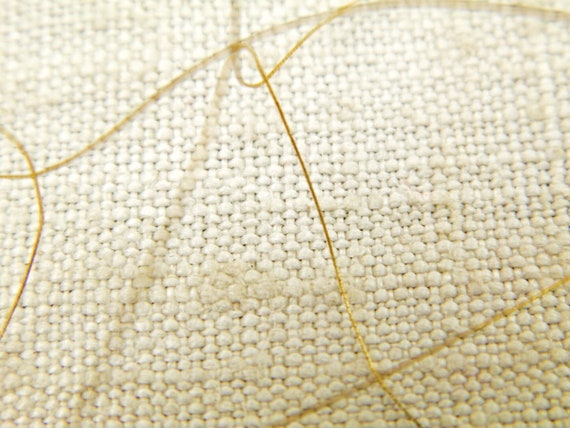This image is a detailed close-up of a woven material, primarily cream-colored, resembling the texture and appearance of a placemat commonly found on a dinner table. The weave is composed of thick white or off-white threads that vary in width, creating a pattern where some areas are wider and others are narrower, suggesting a semi-random weaving method. The overall stitching is somewhat loose, giving the material a relaxed texture. Overlaying this woven fabric are thin golden threads that appear to be casually placed or dropped, forming an informal, crisscrossing pattern. These golden strings create a subtle, uneven checkerboard effect, although the close-up nature of the photo only reveals a few squares of this pattern. The woven material transitions from an off-white at the bottom to a brighter white towards the top, enhancing the textual depth and complexity of the fabric.